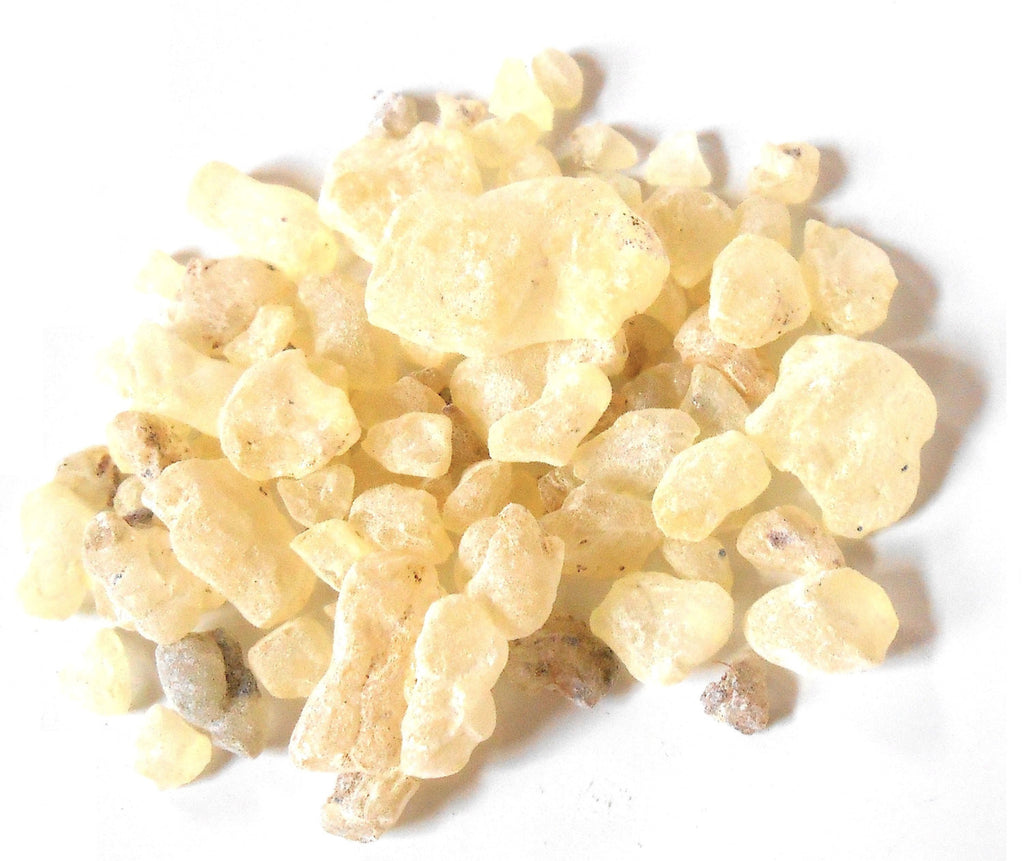This photograph presents a close-up view of a small pile of irregularly shaped, yellowish particles on a white background, resembling pebbles or pieces of dried fruit. The particles, roughly comparable in size to pebbles one might find in a riverbed, vary in color from a bright, cheerful yellow to a more muted, dusky brown-yellow. They have a powdery, unsmooth exterior speckled with tiny occlusions and spots of black and brown. The composition features the largest pieces prominently in the upper center and right center of the image, both casting dark gray shadows on the right and slightly below. The pieces are marbled in appearance, suggesting a certain translucency or coating, reminiscent of dried ginger or solidified honey. The diverse shapes and sizes add to the texture and complexity of the pile, giving it an intriguing, scientific, or experimental quality.